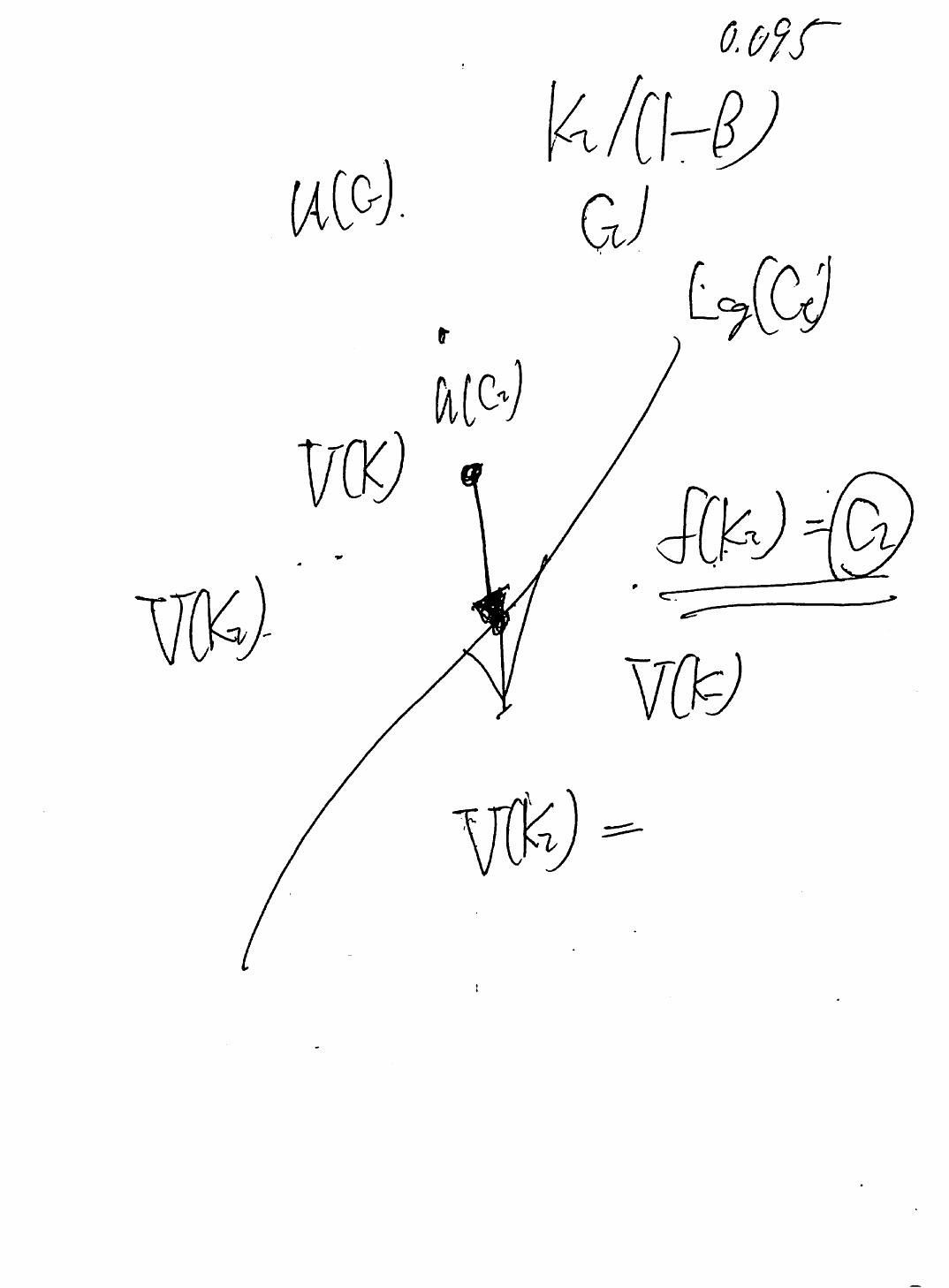The image showcases a linear graph drawn in black ink on a white background, depicting a straight line ascending from the lower left to the upper right, indicating a positive slope. In the center of the line, there is an arrow pointing perpendicularly to the middle of the line. Surrounding the graph are various formulas that appear to be from the fields of chemistry or physics. Notable among these are "V(k2) = ..." and "k2 / (1 - β)", suggesting an attempt to solve a complex equation. The overall impression is of a detailed and technical scientific analysis in progress.